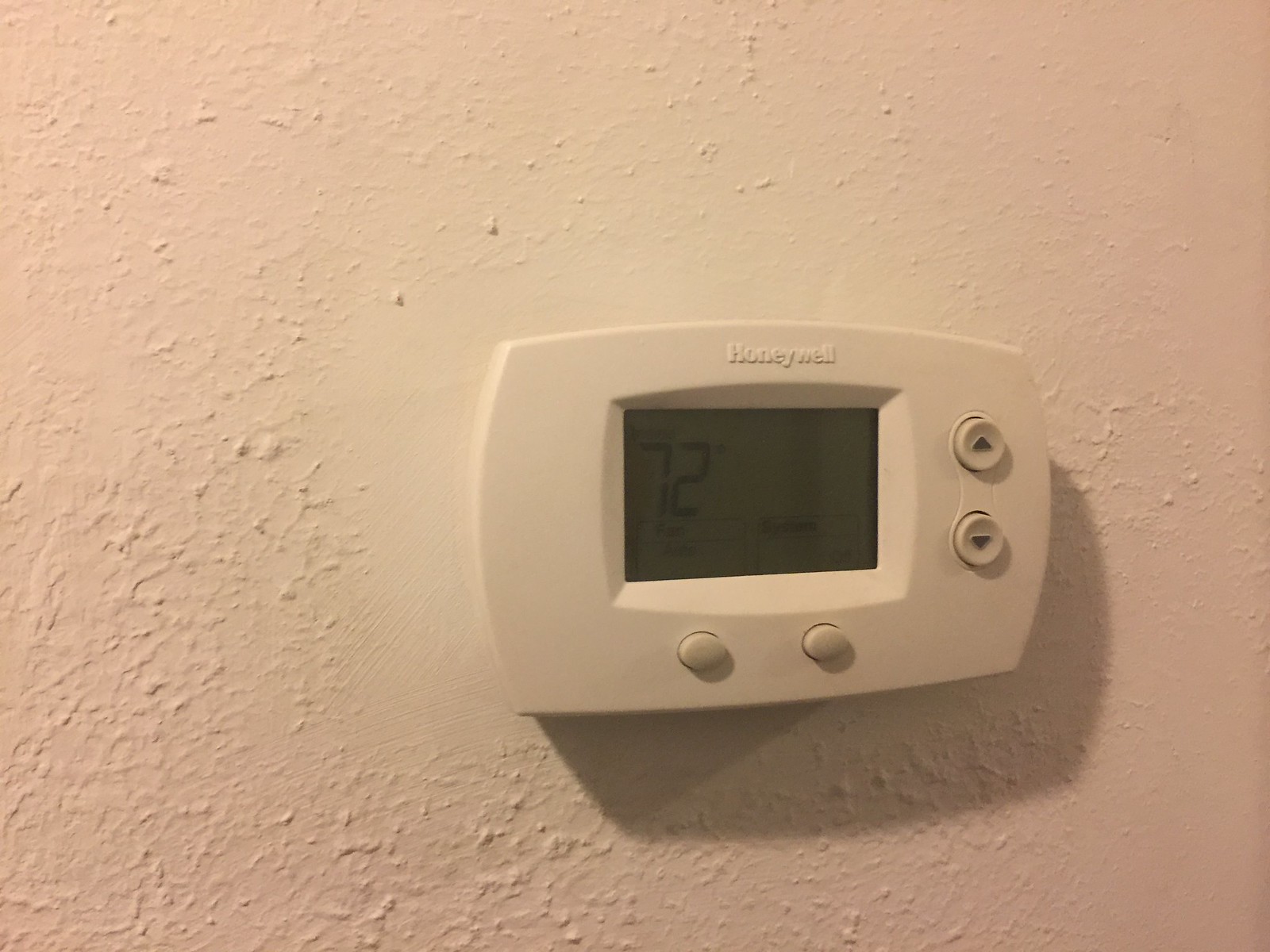The photograph, presented in landscape format and in full color, captures a textured white wall, its surface marked by notable granularity and an uneven finish. At the center of the image, the wall appears to have been sanded smooth, creating a flatter, more polished area. 

Mounted on this smoothed segment is a white plastic thermostat, commanding immediate attention. The thermostat exhibits an ovular shape with a central rectangular digital screen displaying the temperature reading, "72°F." Surrounding the display are various controls, including up and down buttons and additional function buttons beneath, likely used to adjust and regulate the heating settings.

Lighting in the scene originates from the top left, casting a visible shadow on the bottom right side of the thermostat, subtly emphasizing the device's protrusion from the wall. The overall composition highlights the contrast between the textured wall and the sleekness of the thermostat, accentuated further by the play of light and shadow.